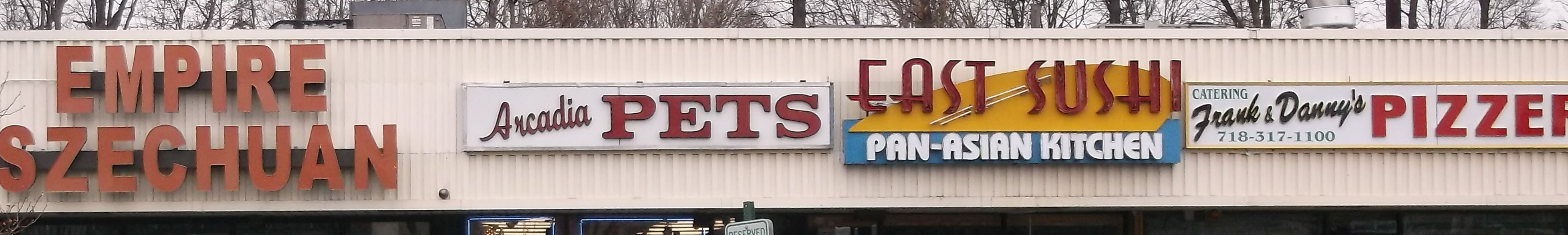This image captures the exterior of a strip shopping center, showcasing various business signs against a backdrop of blue sky with some clouds. The building features cream-colored metal paneling and a mix of ventilation units on the roof. Prominently displayed, the first sign reads "Empire Szechuan" in bold red letters, supported by dark beams. Adjacent to this, a smaller sign with a white background and red text says "Arcadia Pets." Further right, a colorful sign for "East Sushi" features an illustration of a sun, bowl, and chopsticks, with the phrase "Pan Asian Kitchen" in white letters below. The final sign in the sequence advertises "Frank and Danny's Pizzeria" with a cream border, listing a phone number, "718-317-1100," and the word "Pizzeria" partially visible. Trees with varying foliage, some with brown leaves and others bare, can be seen in the background.